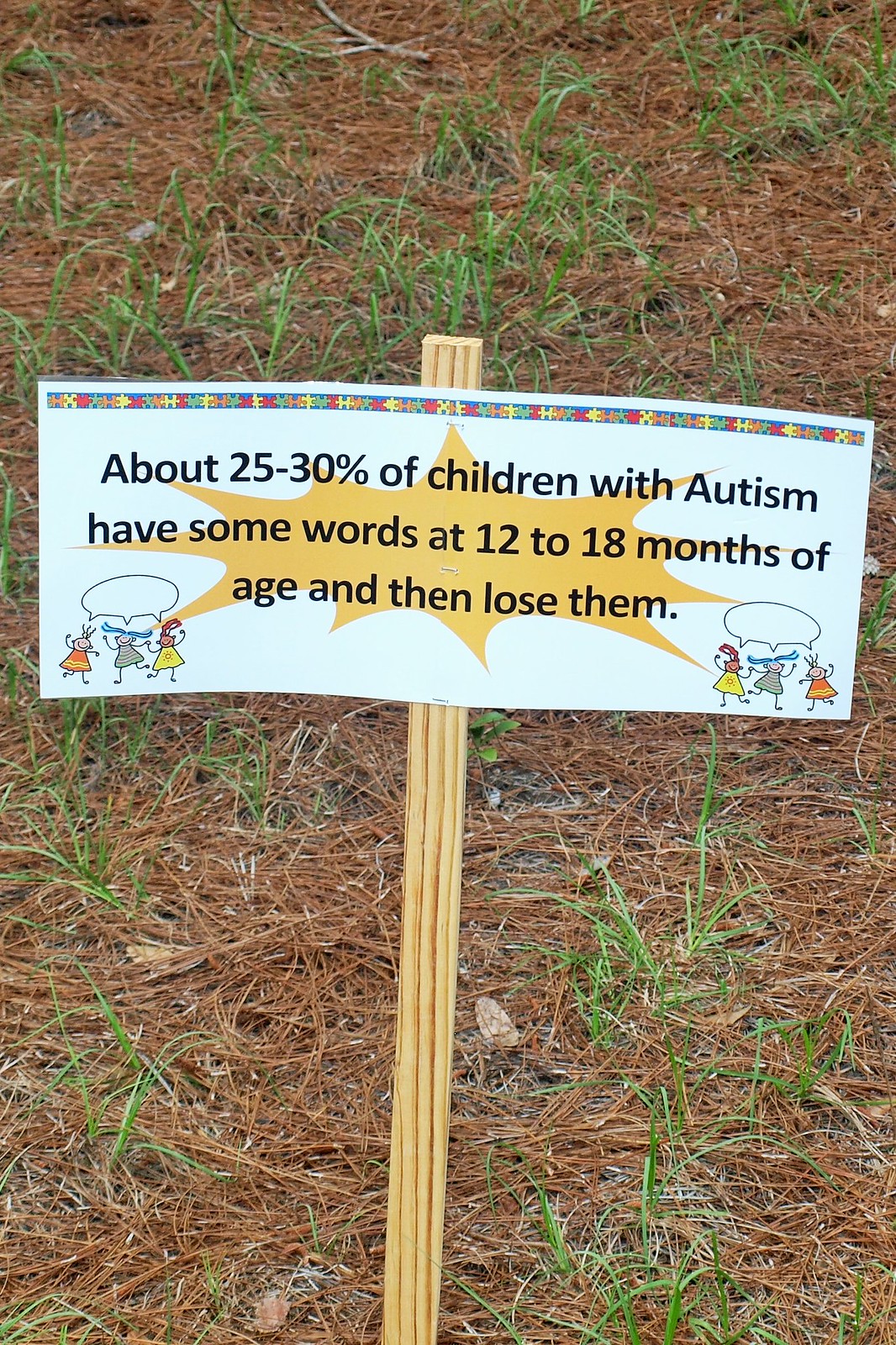The photograph depicts a rectangular white signboard attached to a wooden stake, placed on the ground covered with a mix of green grass, brown grass, dead pine needles, and scattered sticks. The wooden stake supporting the sign appears to be light yellowish-brown. The text on the sign, written in black sans-serif font, reads: "About 25-30% of children with autism have some words at 12-18 months of age and then lose them." The bottom corners of the sign are adorned with drawings of cartoon children, each accompanied by empty speech bubbles. Additionally, a line of puzzle pieces decorates the top of the sign, enhancing the visual appeal and emphasizing the message about autism.